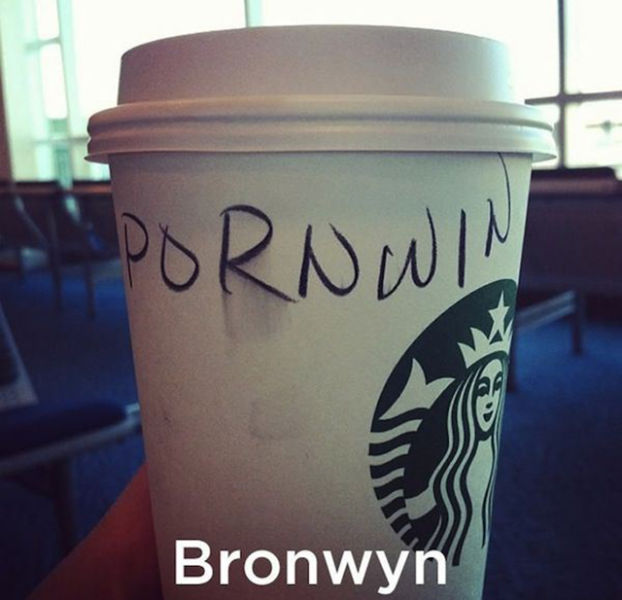The photograph depicts a close-up of a white Starbucks coffee cup featuring the iconic dark green mermaid logo on the right side. The cup is being held by a person in what appears to be a well-lit indoor space, potentially a Starbucks café, identifiable by the blue floor, seats, and windows in the background. Handwritten on the cup in black ink, the name "PORNWIN" is visible, with the poorly written "R" notably smudged, indicating it was done while the ink was still wet. Beneath this, in a neatly printed computer font, the text reads "BRONWIN," suggesting a humorous misspelling of the customer's name, "Bronwyn." This amusing contrast between the intended name and the mistakenly written one adds a layer of levity to the image.